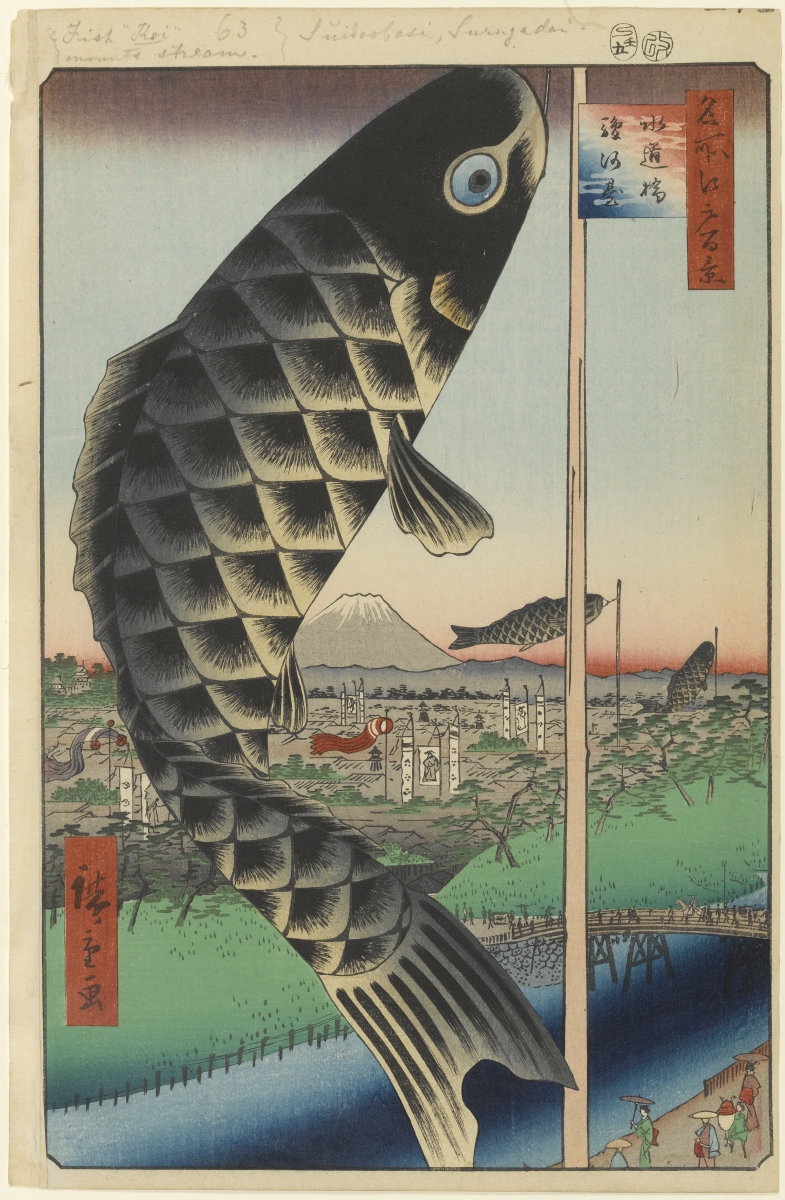This image resembles a tall playing card with a white border featuring beveled edges, and has handwritten notes in pencil along the top border, which read "fish (Koi), number 63." Further down, the barely legible notes mention words like "stream" and possibly "Indonesia" with the term "SURNAJADA." The central focus of the card is a large black and gray koi fish with a blue eye, intricately detailed with large scales, a prominent dorsal fin, and flowing side fins and tail. The fish’s body winds from the bottom middle, curving upwards to the left and then back to the right, with its head at the top middle of the card. In the distance, two smaller fish of the same kind can be seen.

On the right side of the card, a vertically positioned pole spans from the top to the bottom of the image, adorned with a flag at the top. Below the flag is a red rectangle with Japanese writing, arranged vertically. The background features a river flowing from the lower right corner, crossed by a bridge where people are walking. By the riverside in the lower right-hand corner, more people are visible. On the far side of the river, there's green grass, a sandy area with buildings, and in the remote background, a volcano, likely Mount Fuji, is visible. The overall scene captures a blend of aquatic life and scenic landscape.